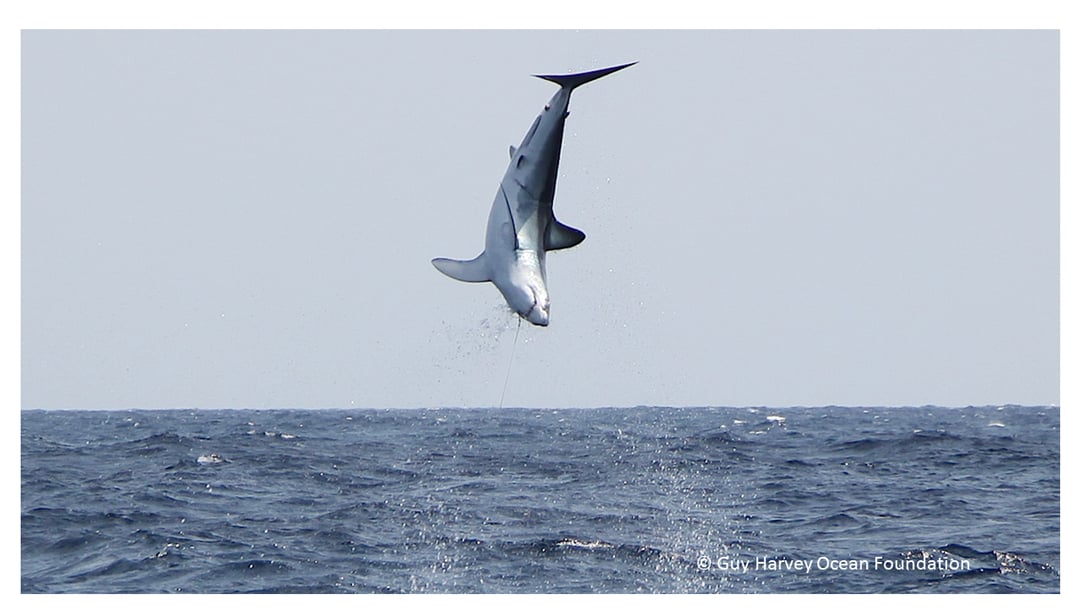The photograph features a dynamic ocean scene with a large shark, possibly a great white, prominently displayed mid-air, diving back into the ocean. The shark's dark gray to black upper body contrasts sharply with its nearly white underbelly. The distinction is vivid as the bottom fades to a lighter gray towards the top. Around the shark, water is splashing energetically, creating a frothy white halo. The ocean beneath is a deep, rich blue, punctuated by darker and lighter patches where the water churns violently. Above, the sky stretches out in a pristine light blue, unblemished by clouds, setting a serene backdrop. The image also has a professional touch, indicated by the white text in the bottom right corner: a circled 'C' followed by “Guy Harvey Ocean Foundation,” confirming its source. The clarity and composition highlight both the shark’s powerful leap and the tranquil yet vast expanse of the ocean, captured in a horizontally oriented frame.